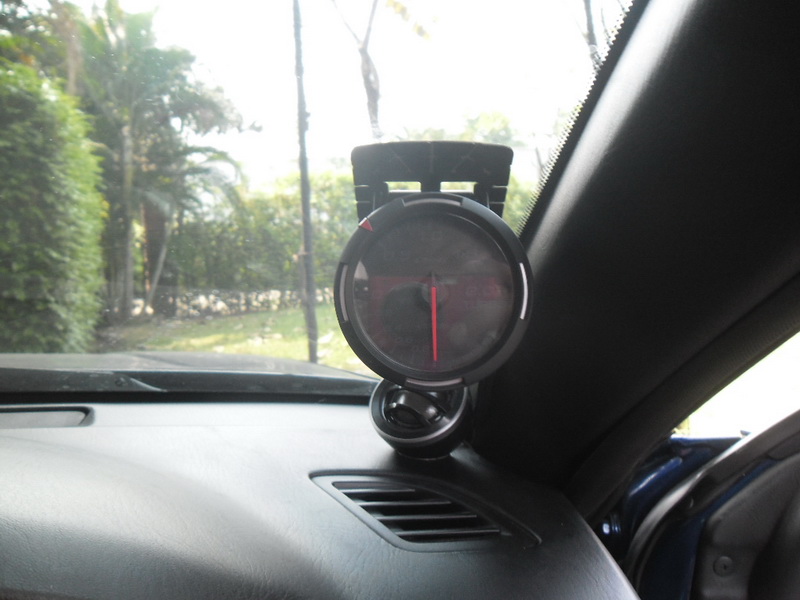Interior scene of a vehicle, presumed to be a police car, with a black dashboard and black interior. Mounted on the dashboard is a black plastic holder typically used for phones, but in this instance holding a round device. The device appears to be a compass with a black and red interior, featuring various numbers around its circumference which are not clearly visible. A red arrow and a red needle are also present on the compass, suggesting directional orientation. 

Outside the vehicle, the scene appears tropical, characterized by at least one visible palm tree and abundant lush greenery. A stone wall is also discernible, possibly indicating a park or natural reserve area nearby, with low grass and several poles resembling dead or bamboo trees adding to the exotic ambiance.

The compass needle is pointing downward, which might imply a misalignment with the presumed north-indicating red arrow. This potential indication suggests the vehicle could be oriented in the wrong direction if navigating by the compass.